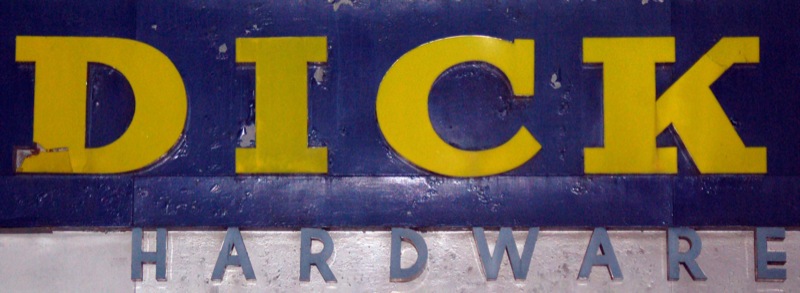In this close-up shot, we focus exclusively on a vintage sign that reads "Dirk Hardware." The sign is distinctly divided into two sections: the upper half is painted a vibrant blue with bold, yellow letters spelling out "Dirk," while the lower section features a silvery-white background with dark blue letters stating "Hardware." Each letter appears three-dimensional, suggesting they were either carved out or meticulously crafted and affixed to the sign's surface. The sign's age is evident, with patches of paint visibly chipping away, lending a worn and nostalgic feel to the image. Due to the zoomed-in nature of the photo, no additional context or surroundings are visible.